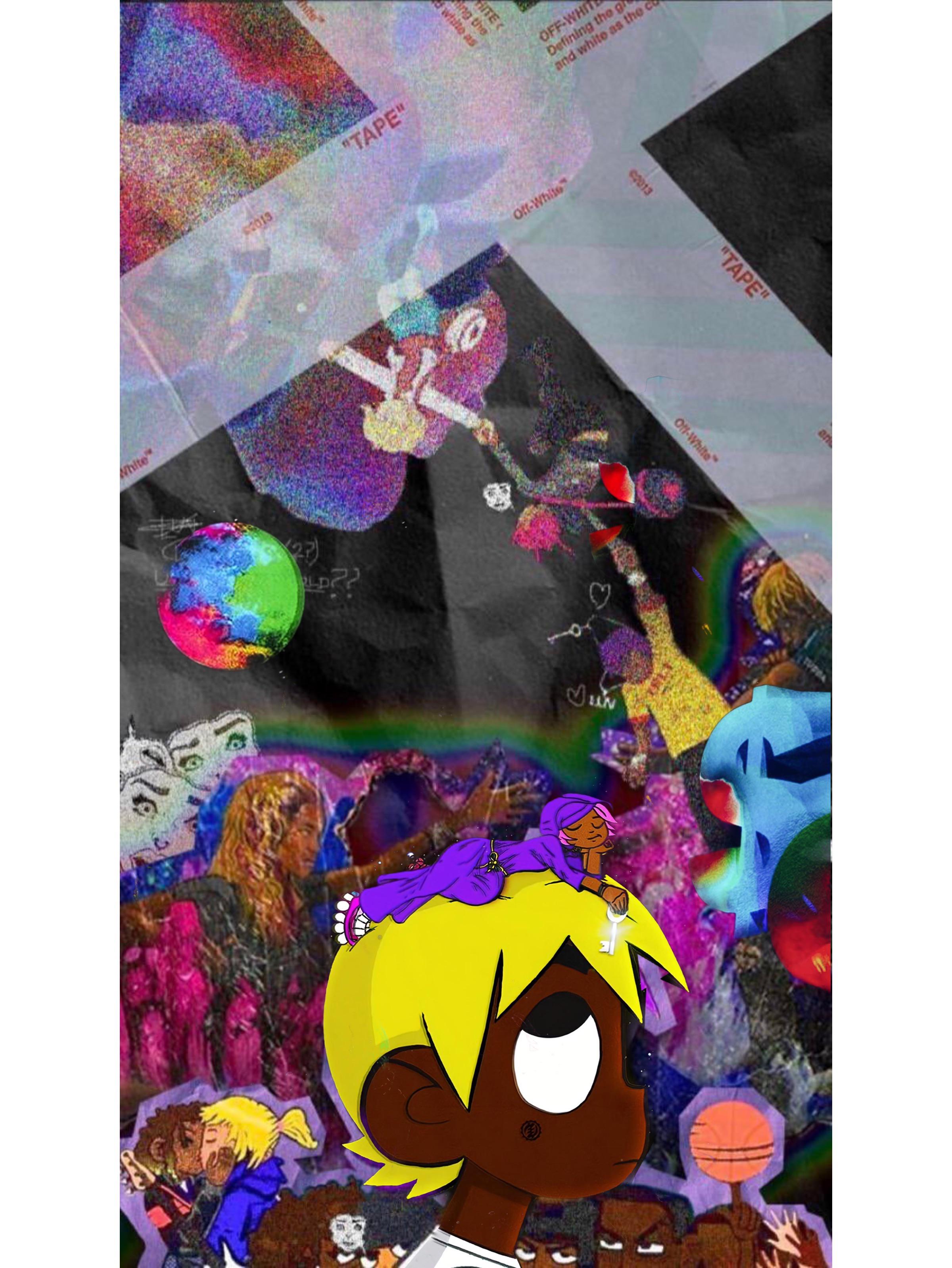The image is a detailed, busy cartoon illustration that is vertically oriented, reminiscent of looking at a smartphone screen in portrait mode. At the top of the image, two pieces of white tape form a cross, with the word "tape" written in red. Below this tape, a vibrant and chaotic scene unfolds featuring numerous cartoon characters, the majority of whom are African American. Prominently, at the bottom of the image, there is a dark-skinned boy with large, expressive eyes gazing upward. Perched on his head is a very small girl dressed in all purple attire, including pink shoes with white circular soles, and she holds a key. His hair is adorned with a black-haired woman in a purple cloak featuring pink highlights. To the left of this boy, a blonde-haired girl in a blue jacket is kissing another character with dark skin and curly hair, dressed in a black jacket with a pink stripe. Additionally, behind this main figure, a finger spins an orange basketball. The collage-like composition of this illustration includes numerous other figures, including a few angry men and various other characters engaged in different activities, creating a whirlwind of visual interest and animated energy.